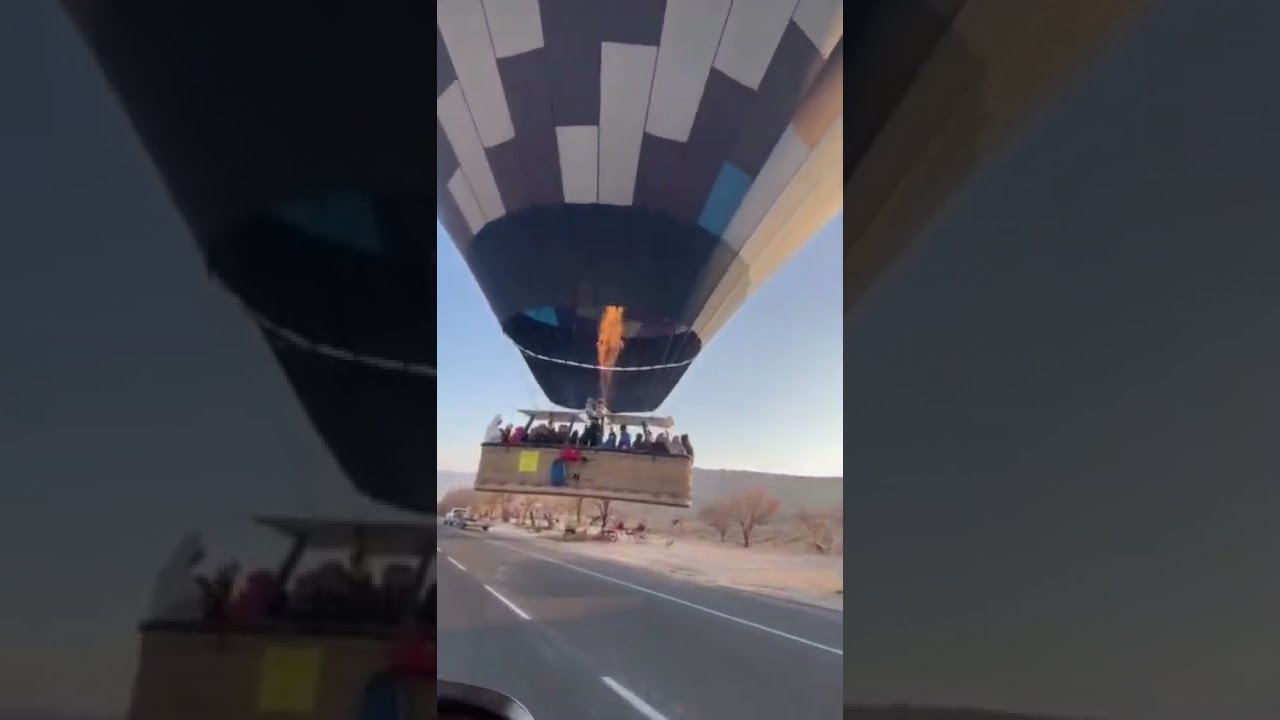A vibrant hot air balloon hovers above a black tarmac highway in a desert landscape, with majestic mountains visible on the horizon under a clear, cloudless sky. The hot air balloon features a striking geometric pattern in black, white, and blue, with an intense orange flame illuminating the inside as it ascends. The gondola basket beneath, constructed of a brownish-gray material, is crowded with a dozen to fifteen excited passengers. The basket is adorned with a neon green square and a blue and red object hanging from its side. A white roof or barrier shields the passengers from the heat of the flame. The scene includes a single car on the road below, and sparse desert flora with brownish leaves scattered around.